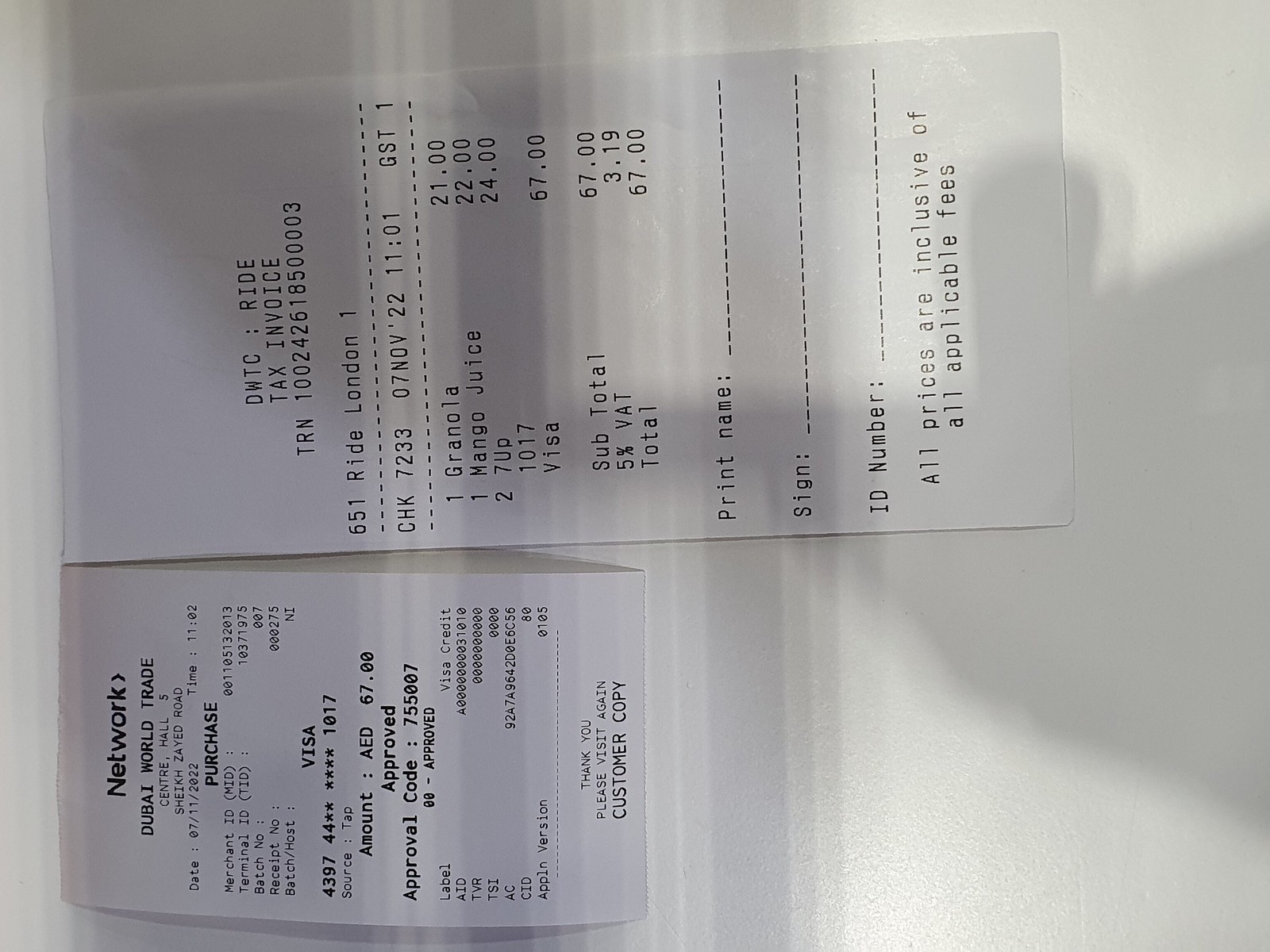The image features two sideways, black-and-white receipts placed side by side on a white surface. Both receipts are printed on white paper with black text. The first, shorter receipt, is from Network Dubai World Trade and shows a purchase amount of $(AED) 67. The text is mostly in dark black, highlighting key sections such as "Network Dubai World Trade," "07/11/2022," "Purchase," and the approval note for a Visa transaction, ending with, "Thank you, please visit again - customer copy." The second, longer receipt is a detailed printout titled "DWTC Ride Tax Invoice," listing items such as granola, mango juice, and 7-Up, and specifying a ride in London. This receipt also shows a transaction approval for AED 67 with additional details, including 5% VAT amounting to 3.19, and it provides areas for a printed name and signature, which remain unfilled. Both documents prominently display transaction information and have areas denoting them as customer copies.